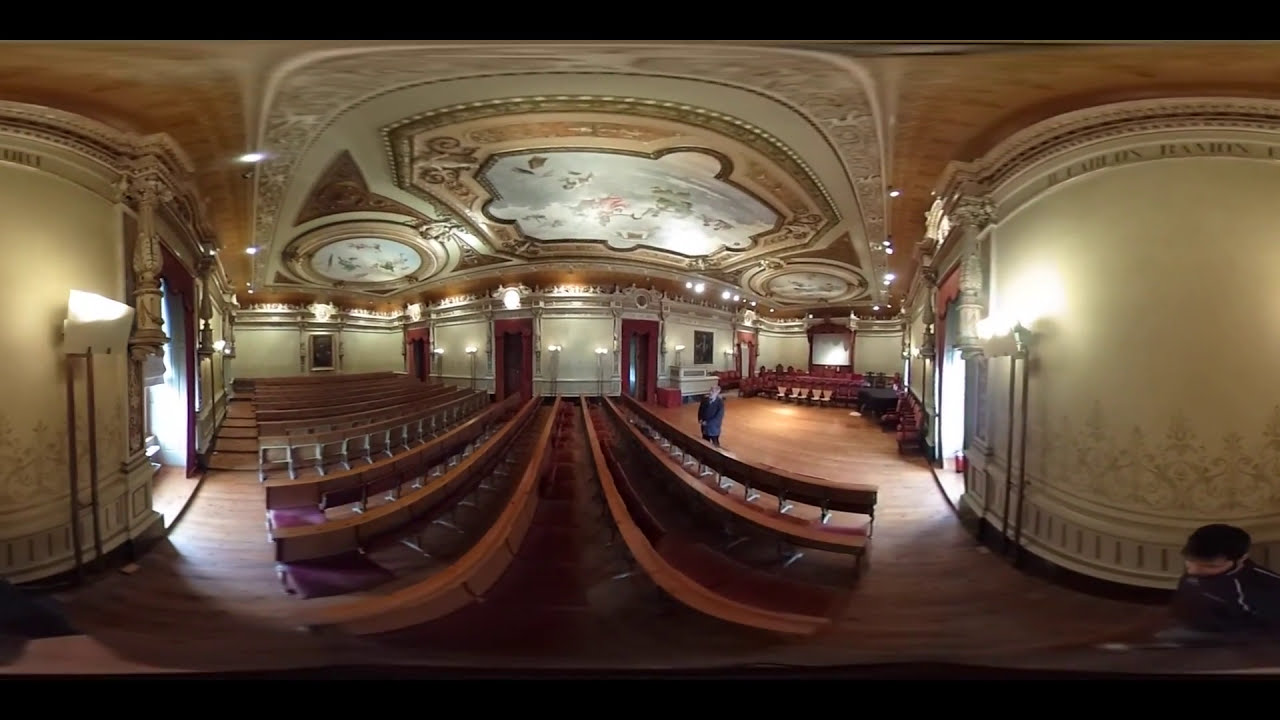The image is a wide rectangular panorama of what appears to be the interior of a vintage performance room or theater, possibly set in a church. The composition has been slightly distorted, bending the straight lines into curved ones due to the camera's panoramic effect.

Starting with the flooring, it features a solid, dark wood floor running down the center aisle, flanked by lighter wooden barriers on either side. The benches, which are the backs of pews facing toward the aisle, have brown wooden backs and are cushioned with black or purple seats, arching gently towards the left side of the image. There are additional wooden barriers on the peripheries of the benches, encapsulating the seating area neatly.

The walls of the room are mainly off-white with detailed gold and light etched embellishments at the top and bottom, particularly visible on the side walls. In the background, the walls feature several red curtained doors, punctuated by lights on each side that create a reflective glow on the white surfaces. The light on the left is held by a wooden stake while the one on the right is brighter. These lights flank doors through which a faint white light emanates, suggesting an adjoining space.

Above, the ceiling reveals an intricate oval design adorned with articulate detailing. The central oval, with a dark brown outline and a mix of white and partially gray hues, is surrounded by lighter cream and pale green colors. Additionally, there are decorative objects resembling flying saucers with white and metallic circles near the center of the oval.

All these elements, from the detailed wooden architecture and ornate ceiling to the embellished walls and pews, contribute to a rich, almost baroque aesthetic, hinting at the room's possible function as a historical or sacred performance space.